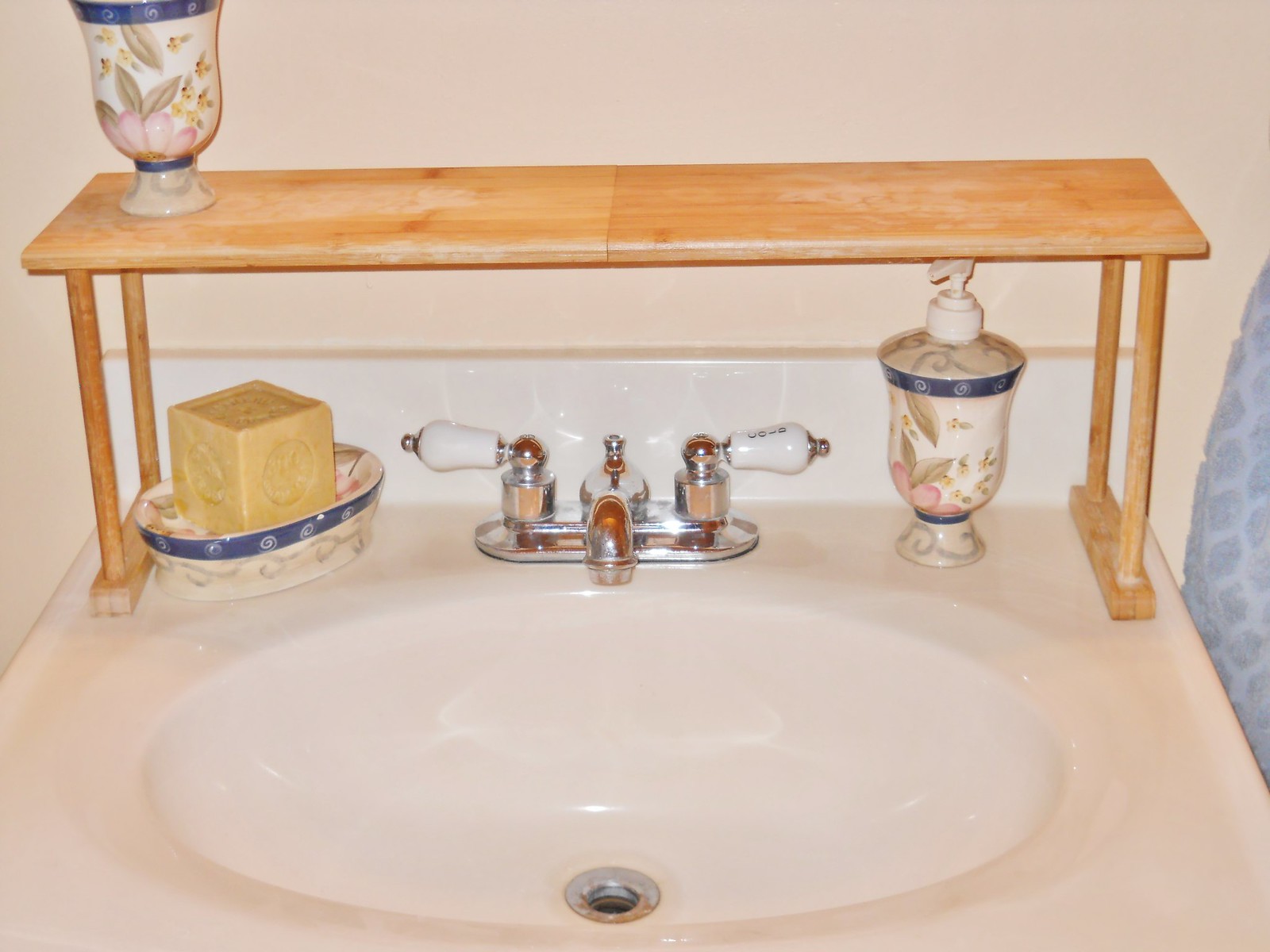A detailed caption for the image described:

The image showcases a stainless steel sink with a gray drainage outlet at the bottom. The sink is equipped with white handles for hot and cold water, with the cold handle positioned on the right and the hot handle on the left. On the left side of the sink, there is a soap holder containing a yellow cube of soap nestled in a white basin. On the right side, a hand soap dispenser is visible. Surrounding the sink are some decorative elements including leaves and an assortment of colors such as pink, blue, and white. Across the center of the sink, a wooden bar extends, adding a rustic touch to the overall setup. In the top left corner, a cup holder is mounted against a beige back wall, contributing to the organized and functional design of the space.